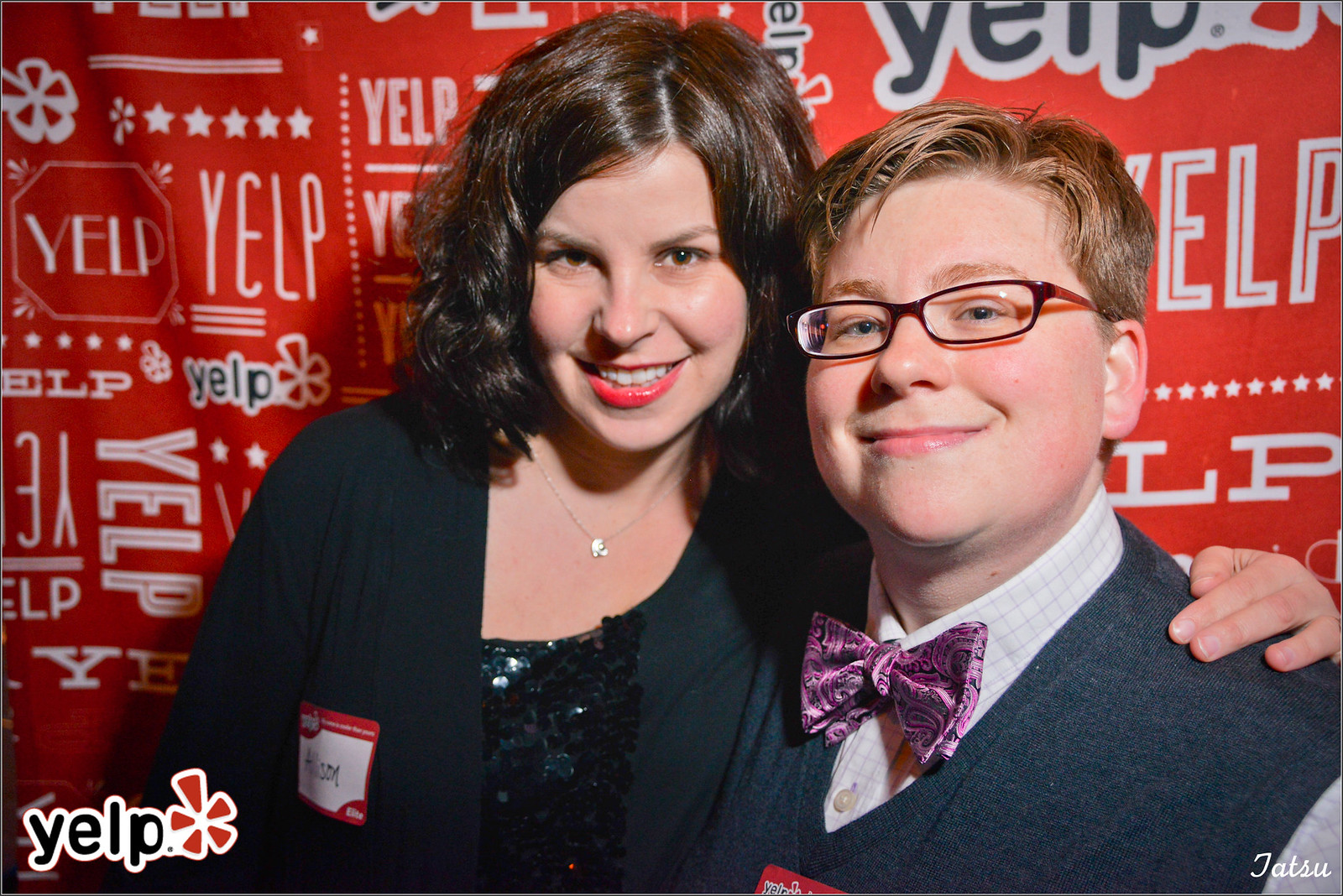This detailed photograph, set indoors, captures a poised pair of women posing in front of a vibrant red backdrop adorned with the repetitive white lettering of "Yelp." The woman on the left, with long black hair and striking red lipstick, appears to be in her twenties. She is wearing a name badge (unreadable) and has draped her arm around the shoulders of her companion. Her outfit consists of a glinty dress beneath a black sweater or jacket, and she accessorizes with a necklace. The woman on the right has short hair, wears glasses, and is dressed in a sharp suit or sport jacket, a checkered shirt, and a distinctive purple bow tie. Both wear name tags associated with Yelp. The bottom left corner prominently features the Yelp wordmark and logo, a black type with a white trim next to a flowery red shape, while the bottom right corner showcases the name "T-A-T-S-U."